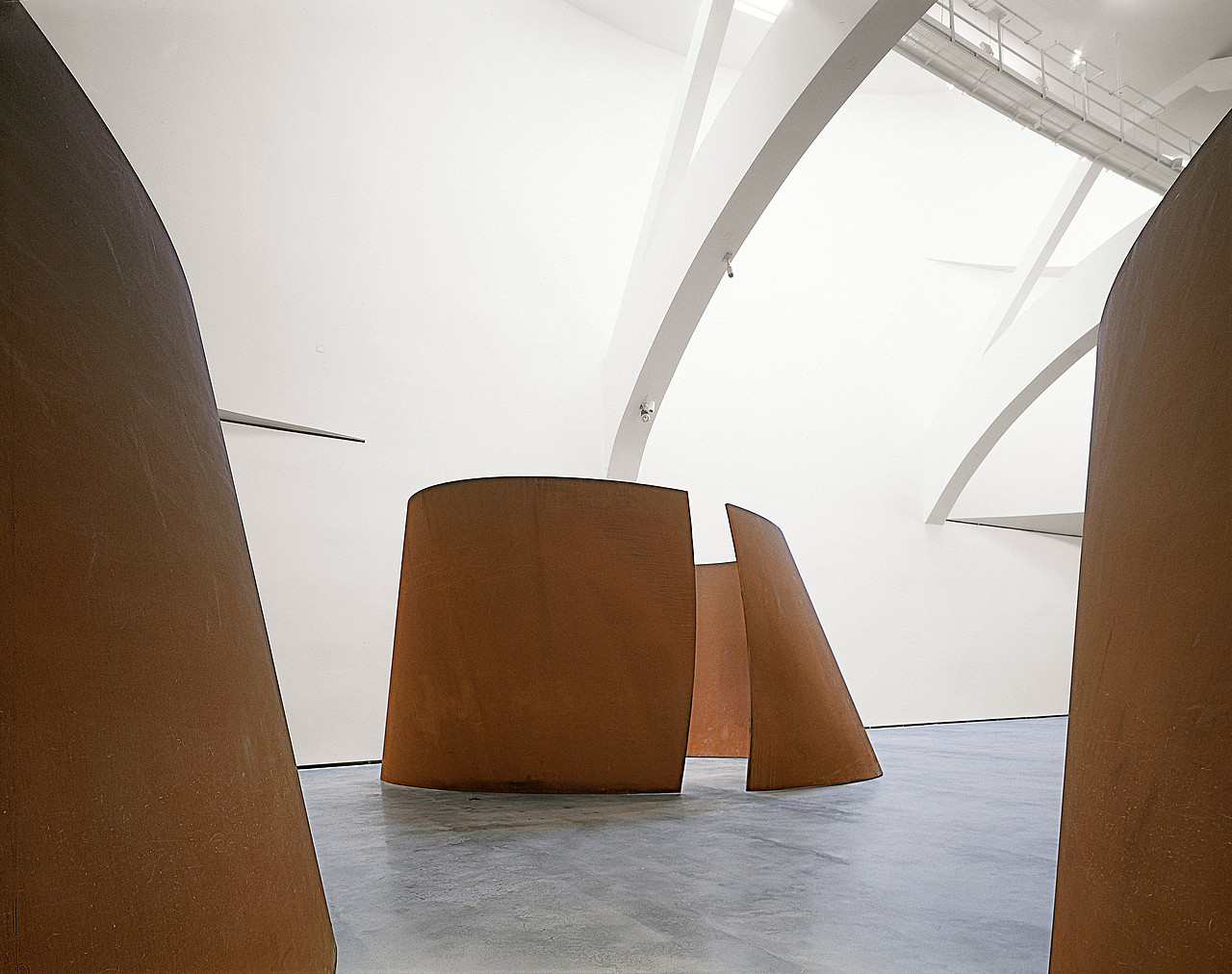The image captures the interior of a large, modern art gallery or installation space characterized by an expansive, curved architecture. The solid white walls rise and curve, supported by white arched beams that add a structural elegance reminiscent of bridge arches. High above on the top right is a white catwalk with a metal guardrail, either part of the gallery infrastructure or a viewing platform.

The floor below is a stark, hard surface with a gray to bluish slate appearance. Standing out against this backdrop are several striking sculptural installations made of thin, orange-tinted material that could be either wood or a thin sheet of steel. These structures are shaped like large, hollow cylinders with openings wide enough to walk through, evoking the appearance of rooms without ceilings or large, curled ribbons creating private enclosures. The central structure is fully visible, showcasing its inviting, open section, while only the sides of two similar pieces are visible at the periphery, suggesting a symmetrical arrangement.

Suspended from the arched beams are what appear to be either cameras or a sprinkler system, hinting at the building's dual purpose of art display and safety. The overall atmosphere is one of modernity and minimalist elegance, punctuated by the intriguing, fluid forms of the sculptural installations.